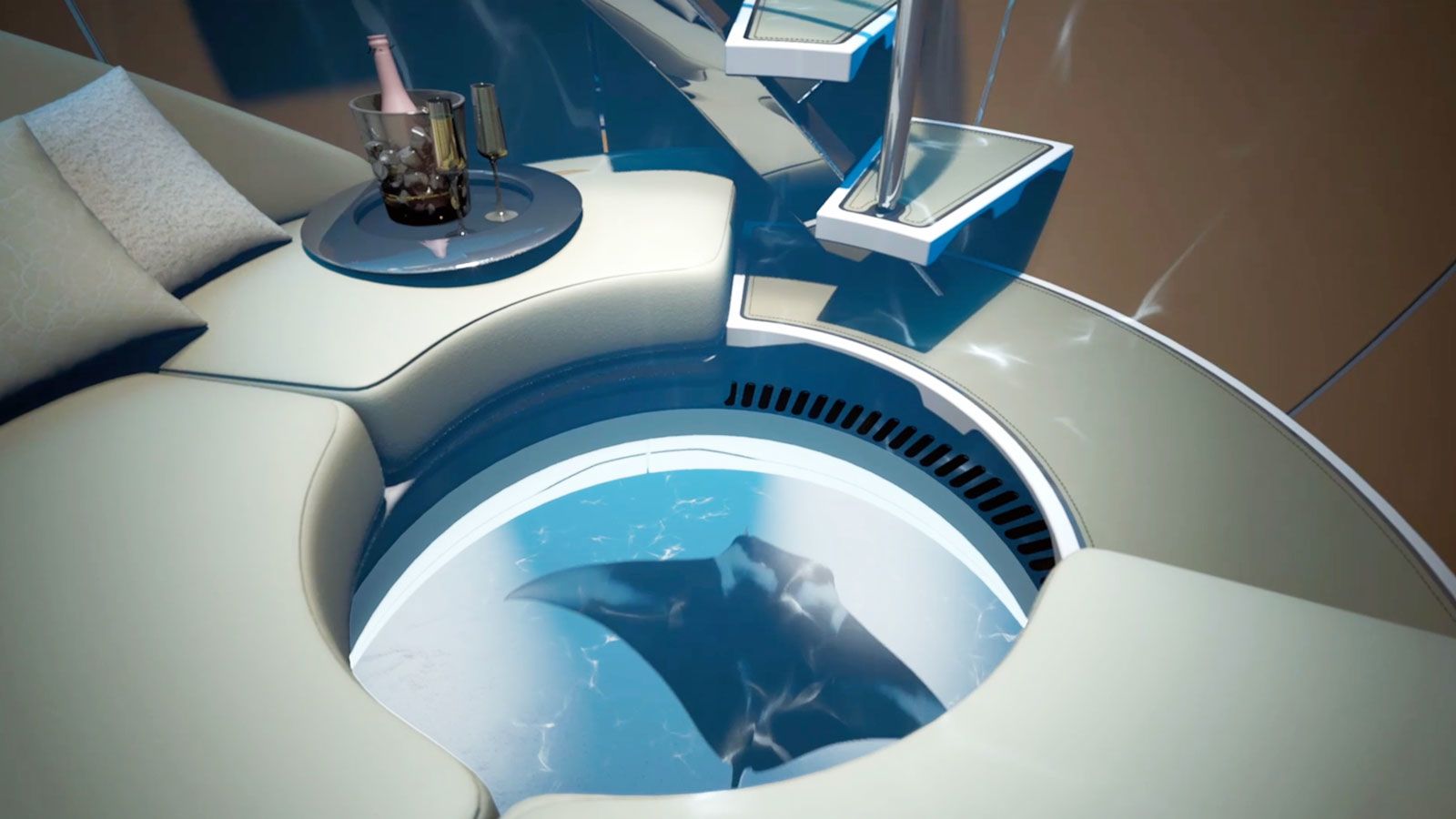This image showcases a modern, circular, white couch with an open section for entry. The seating area is furnished with gray cushions and pillows, forming a cozy nook that surrounds a central glass-covered hole. Visible through the glass, beneath the couch, is a fascinating underwater scene featuring a manta ray swimming. Positioned on the seat cushions is a refined silver tray adorned with an ice bucket containing a pink bottle of champagne and a single champagne flute. In the background, an elegant set of stairs with white outlines, gray central steps, and a silver handrail ascend out of the frame, adding to the chic, contemporary ambiance of the setting. The overall aesthetic of the image is a blend of modern and futuristic design elements.